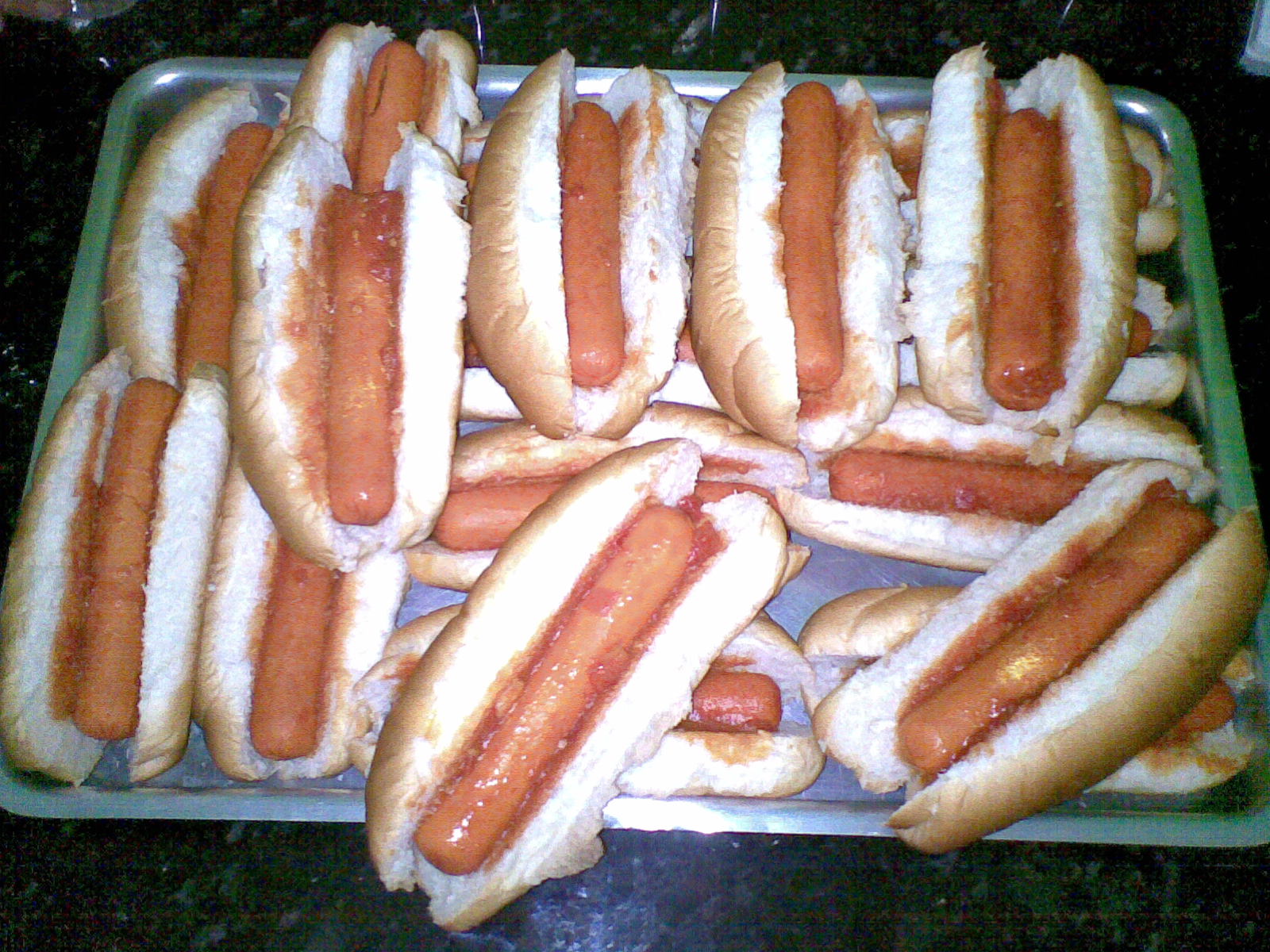The image is a close-up photograph of a rectangular metal tray, primarily silver in color but with some greenish tint around the edges, filled with an abundance of cooked hot dogs nestled in buns. The hot dog buns are golden brown on the outside and white on the inside. Each hot dog is generously topped with vibrant red ketchup. The tray holds more than a dozen hot dogs, scattered in a somewhat chaotic manner; some lie in a straight line, while others are jumbled diagonally or vertically, creating a lively, unarranged appearance. This silver tray is placed on a sleek black marble countertop, enhancing the visual contrast. The hot dogs look fresh, appetizing, and ready to be served.